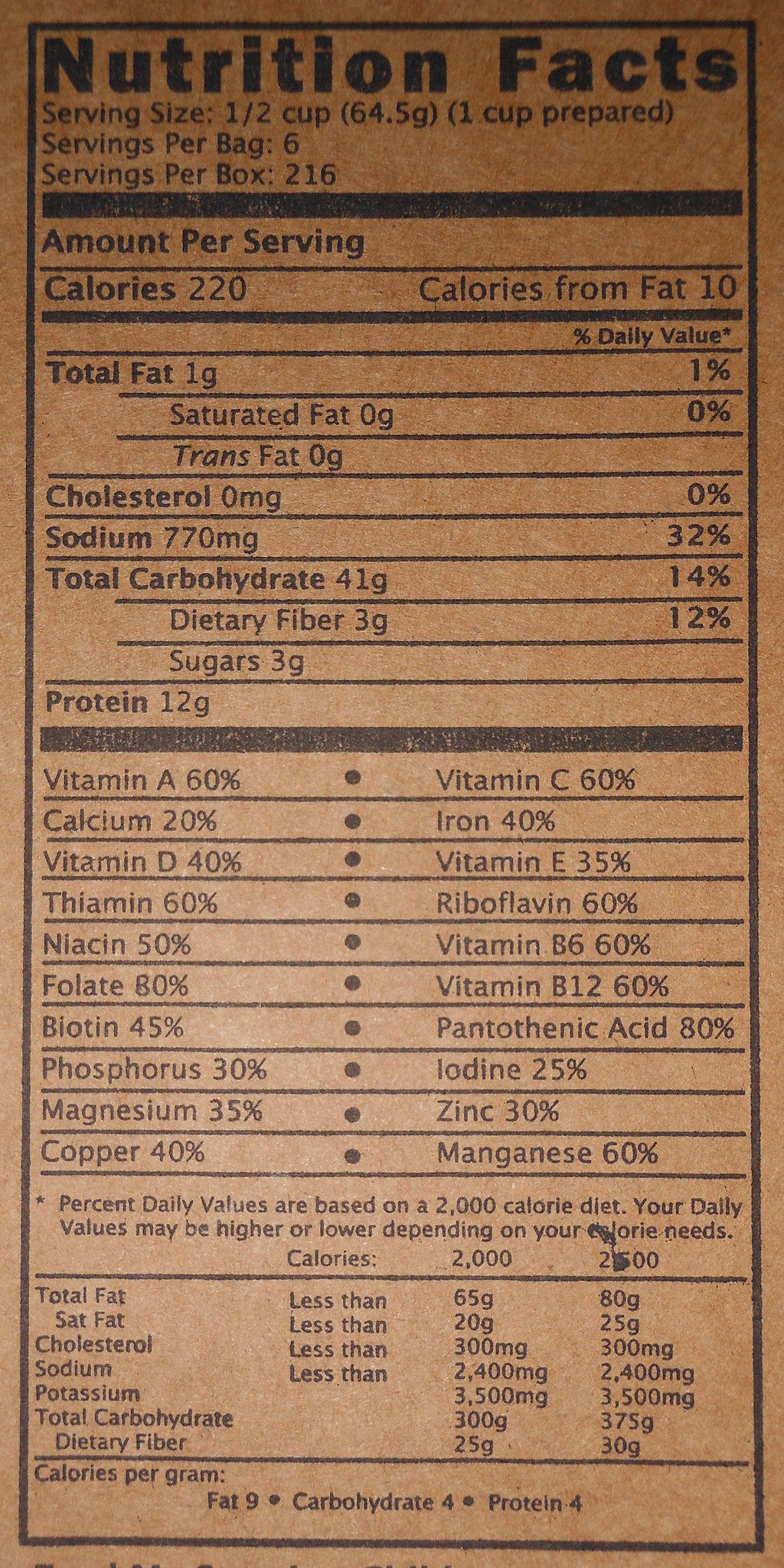This is a photograph of the nutrition facts section from a box of food, possibly cereal or rice. The background of the label is brownish, with all text printed in black. At the top, in large black letters, it reads "Nutrition Facts." The serving size is listed as 1 cup (64.5 grams) when prepared, with 6 servings per bag and 216 servings per box. Each serving contains 220 calories, with 10 calories from fat. 

The label details the nutritional content per serving, which includes 1 gram of total fat, 770 milligrams of sodium, 41 grams of carbohydrates (comprising 3 grams of dietary fiber and 3 grams of sugar), and 12 grams of protein. Cholesterol and trans fat are both absent. 

A black line separates the macronutrient information from the vitamins and minerals section, which lists the daily values for various nutrients: 60% Vitamin A, 60% Vitamin C, 20% Calcium, 40% Iron, 40% Vitamin D, 35% Vitamin E, 60% Thiamin, 60% Riboflavin, 50% Niacin, 60% Vitamin B6, 30% Folate, 60% Vitamin B12, 45% Biotin, 80% Pantothenic Acid, 30% Phosphorus, 25% Iodine, 35% Magnesium, 30% Zinc, 40% Copper, and 60% Manganese. 

At the bottom of the label, it states that the percent daily values are based on a 2,000-calorie diet, with a note indicating that individual nutrient needs may vary. Additionally, it provides a breakdown of calories per gram for fat (9 calories), carbohydrates (4 calories), and protein (4 calories).